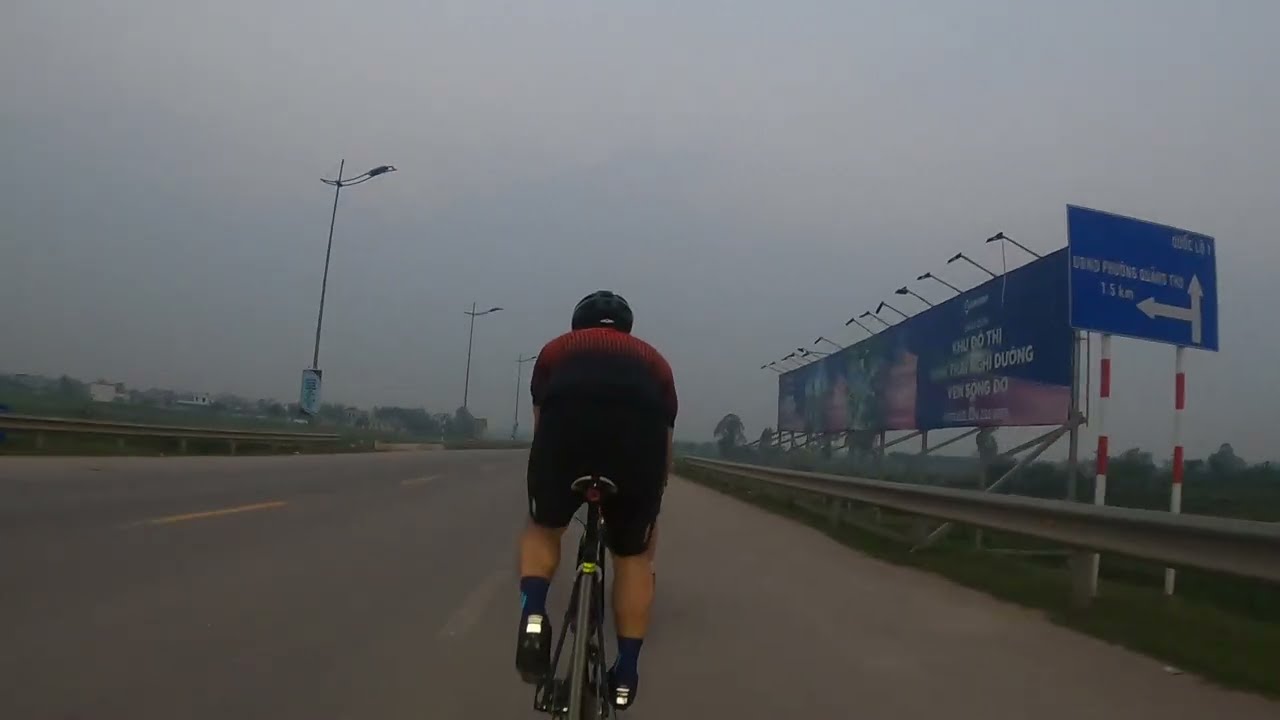The image is a detailed freeze-frame from a GoPro video in landscape orientation, capturing the back of an adult male riding a racing-style bicycle on a multi-lane street or highway. The cyclist, clad in black shorts, blue socks, and a red or burgundy shirt, is slightly hunched over in a typical racing position. His black helmet, along with both feet securely on the pedals, is clearly visible. The scene includes various background elements such as a metal median divider with grass beyond it on the right, along with a large billboard and directional signage in a foreign language. These elements, featuring blue backgrounds with white arrows and red and white posts, signify different city directions. On the left-hand side, the image shows tall streetlights and overhead traffic signals, which are not illuminated. The overcast and cloudy sky adds to the moody ambiance of the photograph, while green trees and bushes provide a natural backdrop. Notably, the road appears devoid of other cyclists or vehicles, implying this is not part of a formal bike race. The photo perfectly captures a moment of solitary cycling adventure on a desolate, urban freeway.